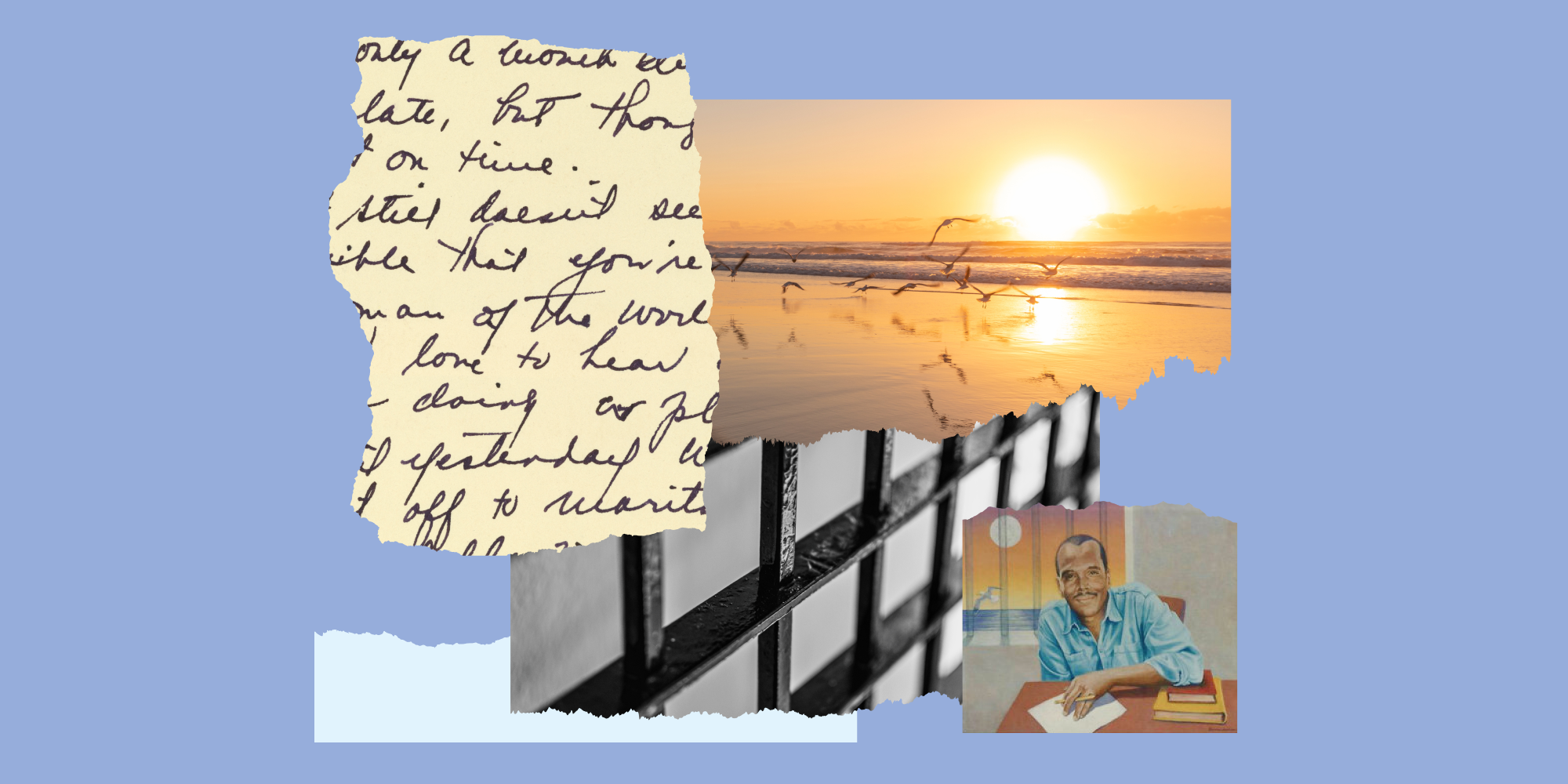The image is a complex digital collage set against a bluish-purple background, integrating several elements to convey a vivid narrative. Central to the collage is a realistically drawn dark-skinned man with a mustache, seated at a desk. He is wearing a blue shirt and holds a pencil in his hand, poised over a white piece of paper, with a book under his arm. The man's setting includes a gray wall behind him, giving the impression of a jail cell, emphasized by an image of black jail cell bars placed to the right. This jail cell imagery is realistic and black, indicating confinement.

Above the man's depiction is a serene photograph of a sunset over a beach, featuring birds in mid-flight above the ocean's shimmering waves, capturing a moment of tranquility and freedom. To the left of the sunset is a torn-out portion of a handwritten note, seemingly in black cursive on a pale yellow background. This note appears fragmented and adds a personal, intimate touch to the composition, even though the text is mostly illegible.

Together, these elements—the realistically drawn incarcerated man, the photographic details of jail bars, the serene beach sunset, and the torn handwritten note—create a rich, layered visual story against a cohesive purple hue, juxtaposing themes of confinement and freedom.